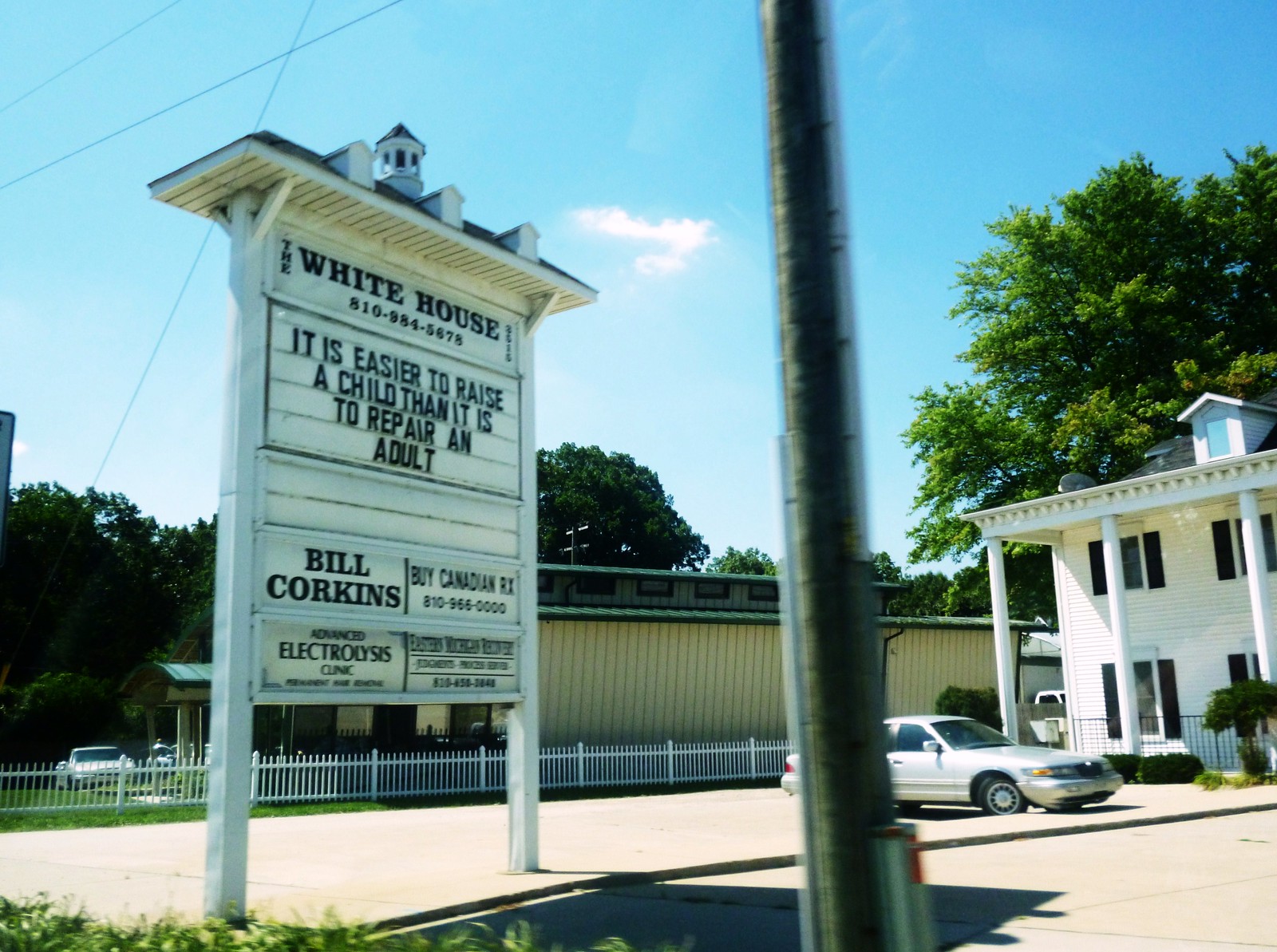The photograph captures a sign situated in a parking lot, presented in a rectangular format with the top and bottom edges being the longer sides. Prominently positioned in the foreground is a wooden telephone pole, adorned with metal gray wire coverings on both its left and right sides, and smaller poles attached at the bottom. To the left of the telephone pole stands a rectangular sign topped with a small slanted roof. The sign comprises several white rectangular sections, each displaying different lines of black text. The text reads, from top to bottom: "The White House, 810-984-578" followed by the quote, "It is easier to raise a child than it is to repair an adult. Bill Corkins," and continues with, "by Canadian RX, 810-966-0808. 810-966-0000."